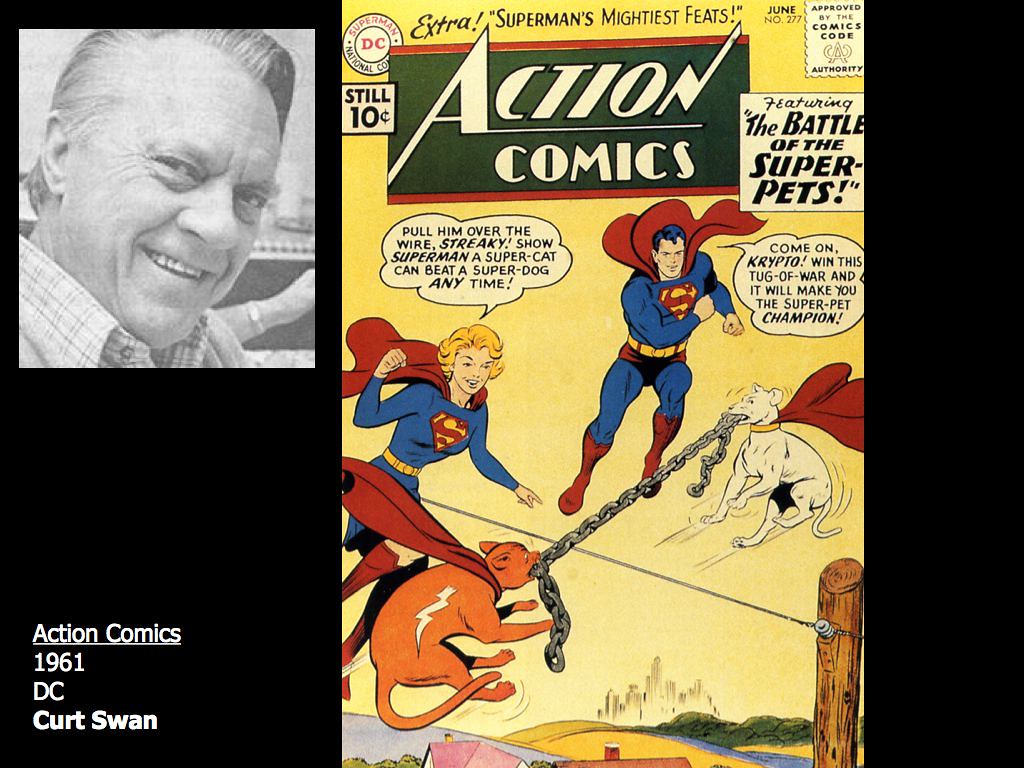The image features the vibrant cover of an old comic book titled "Action Comics," with the issue prominently showcasing "Superman's Mightiest Feats." At the top of the cover, the words "Extra!" are emblazoned in small black print against a yellow background. Below this, the iconic "Action Comics" logo appears in white letters with a black backdrop. The publication date, June 1961, and the price, "still ten cents," are clearly visible, along with the "Approved by the Comics Code Authority" seal. 

In the center of the cover, Superman is depicted flying with his cape billowing behind him. To his right, Superwoman (or possibly Supergirl, based on the descriptions) mirrors his airborne pose. Below them, two dogs, each wearing a red cape, engage in a spirited tug-of-war. The white dog, Krypto, is pulling against a brown dog named Streaky, reinforcing the theme of "The Battle of the Super Pets," which is highlighted on the cover. 

The background of the cover illustrations includes trees, water, dirt, cityscapes with tall skyscrapers, and rooftops from a town below, set against a yellow sky. Additionally, there are dialogue boxes with playful text: "Pull him over the wire, Streaky! Show Superman a super cat can beat a super dog any time," and "Come on Krypto, win this tug-of-war and it will make you the super pet champion."

In the upper left corner, there's a black-and-white illustration of the artist, labeled with "Action Comics 1961, DC, Kurt Swan." This cover art brims with vivid imagery and dynamic action, effectively conveying the excitement and playful competition among the superhero pets.